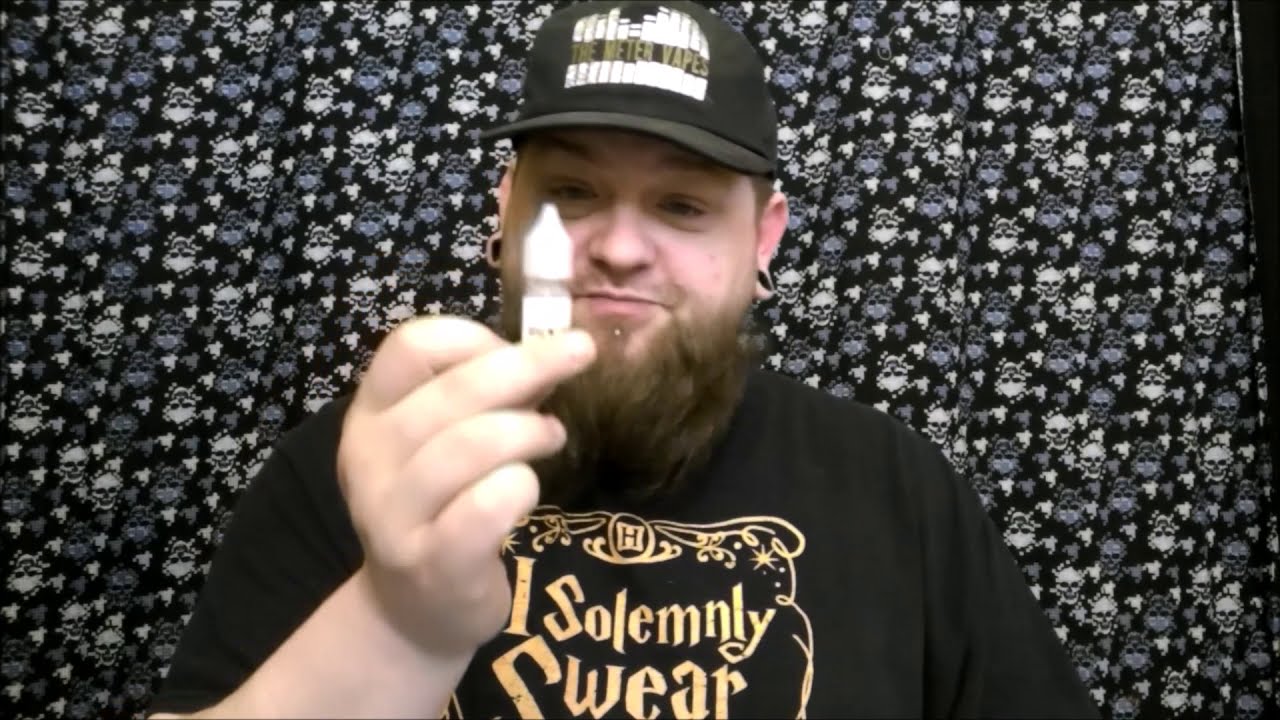The photograph features a larger white man with round cheeks, a prominent, bushy brown beard, and a hint of a mustache. He is wearing a black baseball cap that reads "The Meter Vapes" in red writing with some white markings on it. His outfit includes a black T-shirt with the gold text "I solemnly swear," a recognizable reference to Harry Potter. The man also has gauges in his ears. He is holding up a small bottle with a white cap in his right hand, which is on the left side of the frame, and appears to be examining it. The background displays a black cloth adorned with a pattern of blue and white skulls, adding a slightly eerie but intriguing atmosphere to the scene.